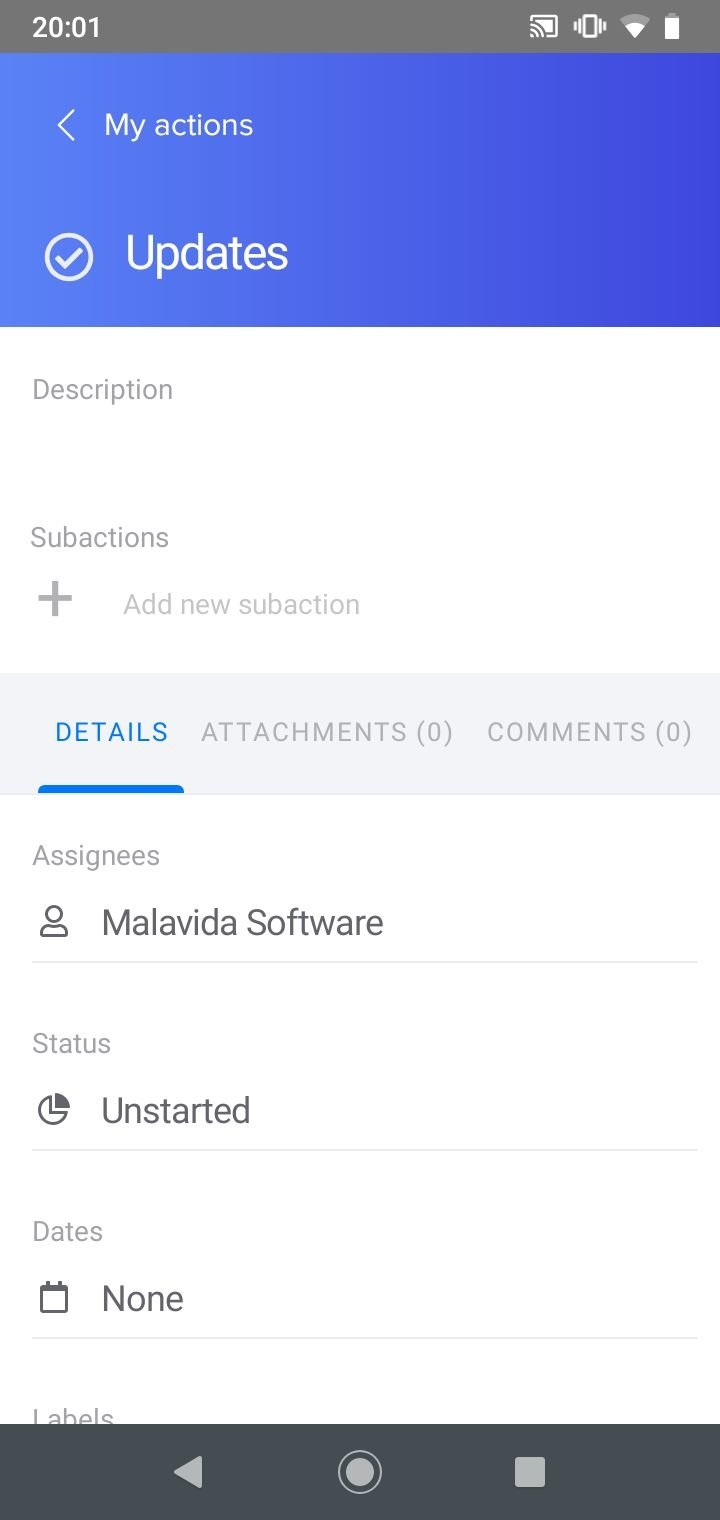This screenshot, taken from a cell phone in portrait mode, captures a user interface screen. In the upper left and upper right corners, the time is displayed as 20:01 against a dark gray background. The next section below features a light blue background. The first row of this section includes a back arrow icon and the label "My Actions." Directly underneath, there's a check mark encased in a circle with the word "Updates" beside it.

The following section appears with a white background. On the left, it reads "Descriptions," and just below this, it states "Sub Actions." Under the "Sub Actions" heading, there is a plus sign icon alongside the text "Add New Sub Actions." 

Proceeding further down, a stripe with a gray background displays three header columns: "Details" (underlined and highlighted in blue), "Attachments 0," and "Comments 0," which remain in gray. Under the "Details" column, the form contains several rows of information:
- Assignees: Molybdenum Software
- Status: Unstarted
- Dates: None
- Labels: (content appears to continue but is cut off in the screenshot)

At the very bottom of the form, there is a black stripe. This stripe includes a back button on the left, a center button featuring a circle, and a gray square icon on the right. The screenshot depicts a form intended for detailing and organizing task or attendance information.